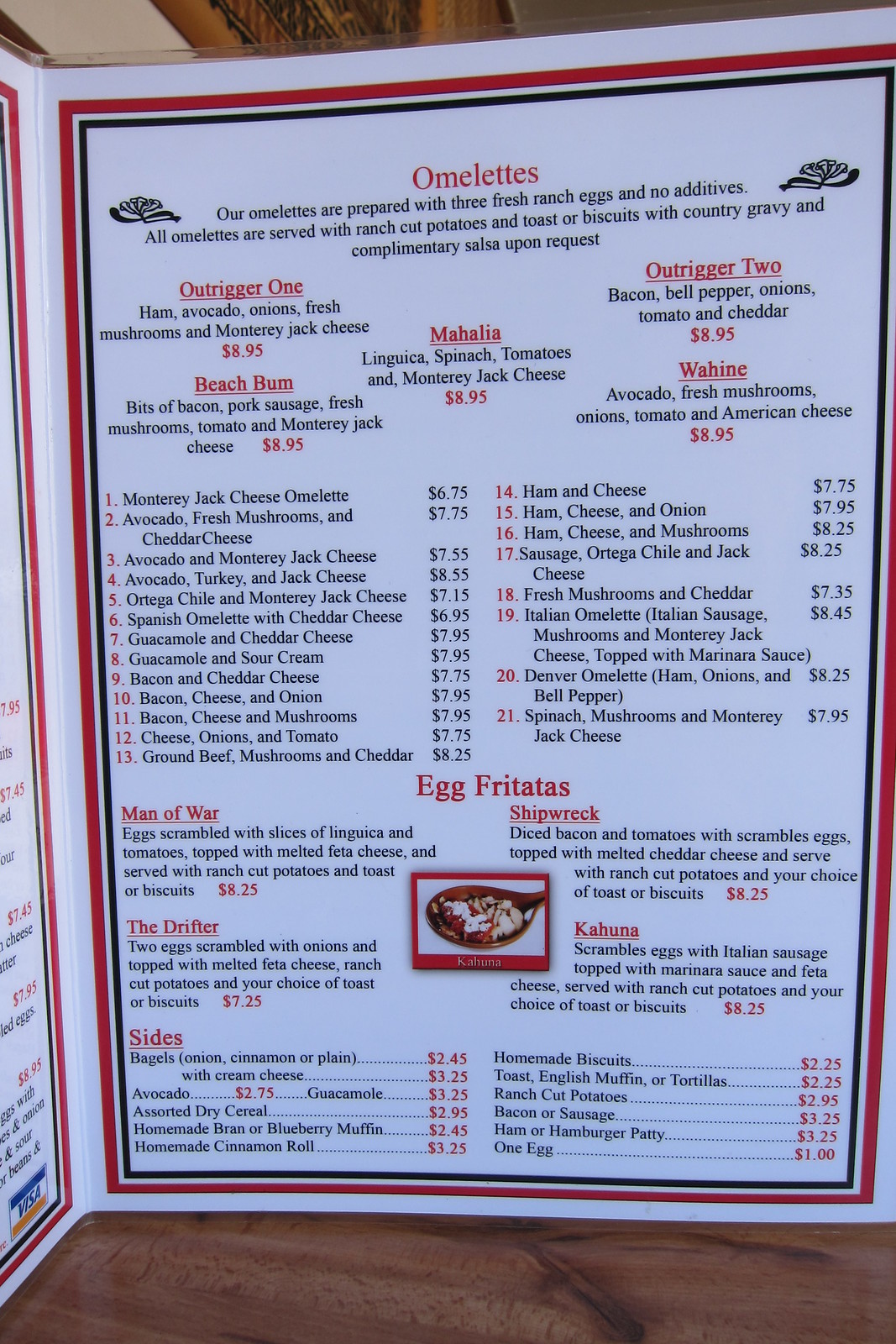A white diner menu stands upright on a wooden table, showcasing a clean and organized presentation. The menu is framed by a red border with a smaller black border inside it. At the top of the menu, two small floret icons add a decorative touch. The bottom third of the menu features an image of the Kahuna, an egg frittata.

The menu's headline reads "Omelets" in bold red letters. Below the title, it states: "Our omelets are prepared with three fresh ranch eggs and no additives. All omelets are served with ranch cut potatoes, toaster biscuits with country gravy, and complimentary salsa upon request."

Five omelets are listed: Outrigger 1, Outrigger 2, Mahalia, Beach Bomb, and Waheen—all priced at $8.95—each accompanied by a detailed list of ingredients. Beneath these, a variety of 21 additional omelet variations are available, with prices ranging from $6.75 to $8.55.

In another red section titled "Egg Frittatas," there are four options: Man of War, Shipwreck, the Drifter, and the Kahuna. All are priced at $8.25, except for the Drifter, which is $7.25. The menu also includes a section for sides, highlighted in red, with all prices listed in the same color except for those in the extensive omelet list.